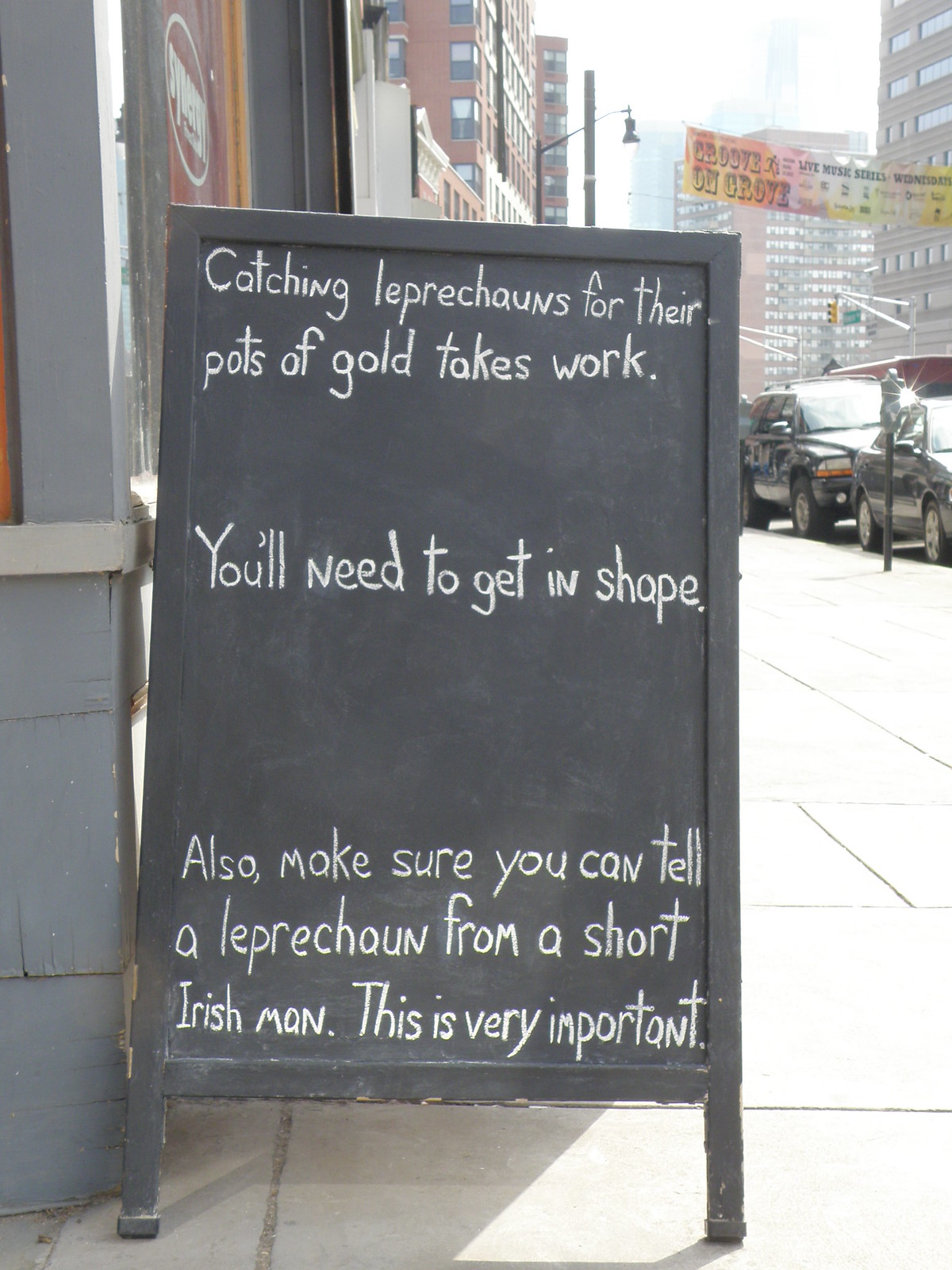In this outdoor daytime photograph set in a downtown city area, the focal point is a black A-frame chalkboard sign positioned centrally on a concrete sidewalk. The sign bears handwritten white chalk text in three distinct sections: at the top, it reads, "Catching leprechauns for their pots of gold takes work." Following a significant gap, the middle section states, "You'll need to get in shape," and at the bottom, it concludes with, "Also make sure you can tell a leprechaun from a short Irishman. This is very important." 

Surrounding the sign are various urban elements: to the left, there's a gray building and a storefront, while in the background, one can see several parked vehicles lined along the street beside parking meters. Further back, there are taller buildings and a banner stretching across the street, although the text on the banner is not discernible. The scene is steeped in urban vibrancy, with colors like tan, gray, light blue, orange, yellow, white, and black visible throughout.